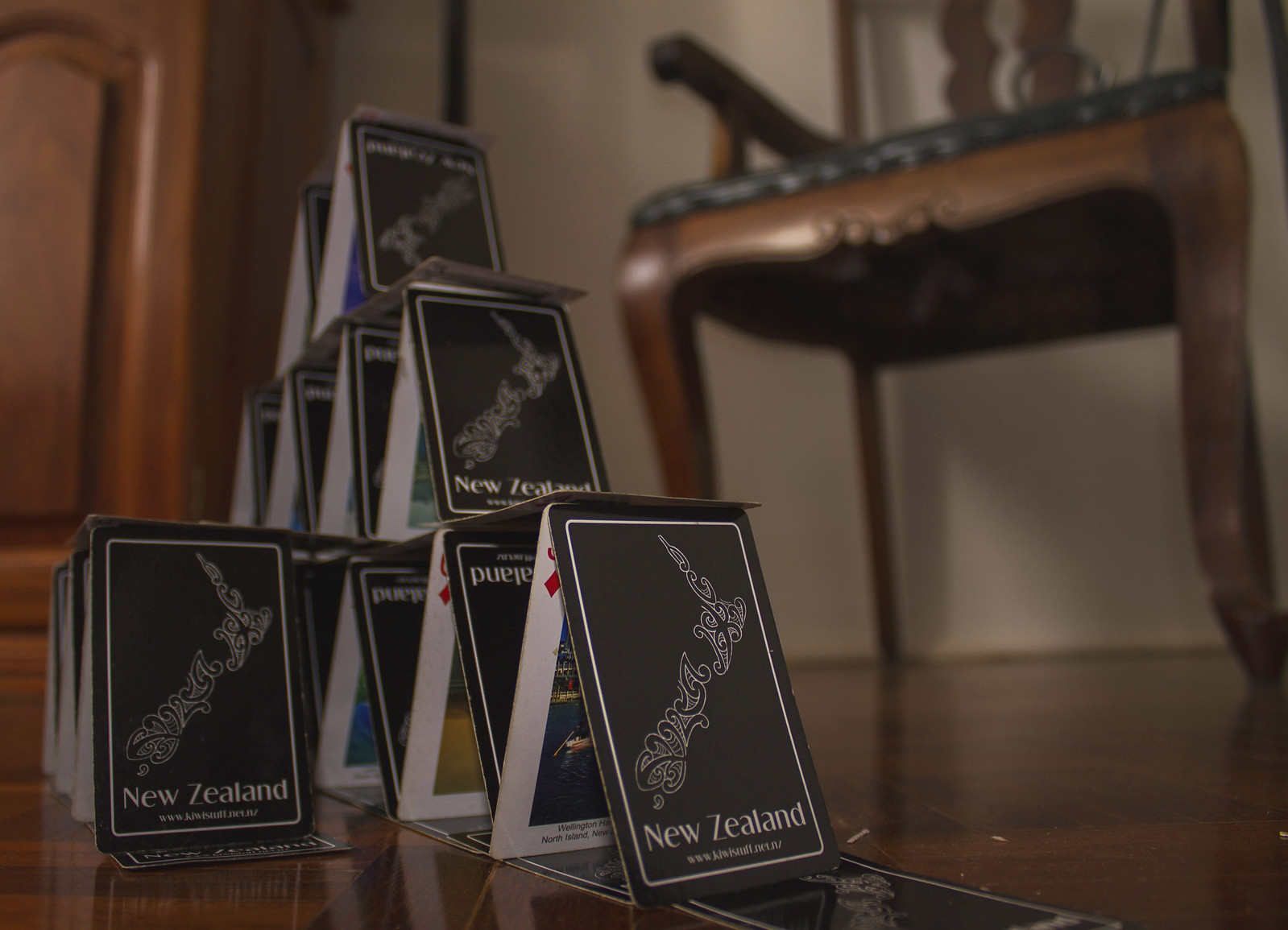This image showcases a meticulously constructed house of cards, arranged in a delicate pyramidal structure. The base layer consists of playing cards laid flat, providing a solid foundation. Two cards, placed upright and leaning against each other, support the next level. Additional cards are arranged in a similar manner along the edges, creating a layered, interlocking formation. Ascending layers of cards continue this pattern, culminating in a pointed peak at the top.

The cards themselves are ordinary playing cards, but the backs feature the word "New Zealand" prominently, set against a black background. The structure stands on a wooden surface that contrasts with the vibrant design of the cards. In the background, there's an old wooden chair, adding a rustic ambiance to the scene. This chair is paired with a full-time chair, hinting at a cozy, lived-in environment. The image captures a moment of stillness and balance, highlighting the fragility and precision of the card pyramid.